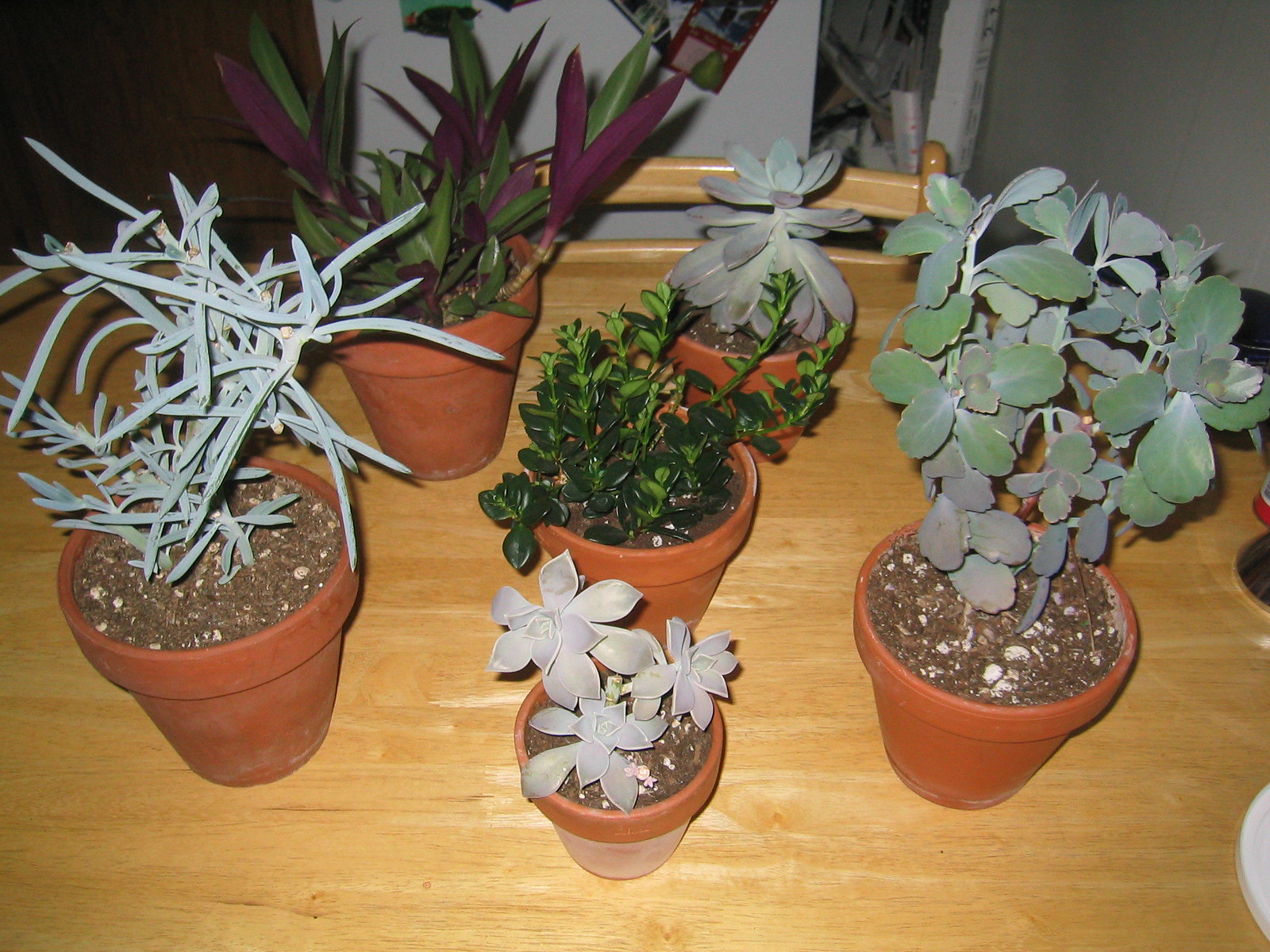This color photograph showcases six potted houseplants, prominently succulents, elegantly displayed on a light brown wooden kitchen table. The plants are housed in classic terracotta pots filled with soil mix, some dotted with white perlite. The arrangement forms a circular pattern around a central plant with dark green, small leaves sprouting from multiple stems.

At the 1 o'clock position, a succulent with lighter green leaves tinged with purplish edges stands out, while the 4 o'clock position features a similar succulent with slightly larger, pale green leaves. A unique succulent at 6 o'clock displays light grayish-green leaves, with hints of lilac. At 8 o'clock, a larger succulent with long, spindly leaves adds height to the ensemble. Finally, the plant at 11 o'clock presents striking purple leaves amidst the varying shades of green.

Behind the plants, a matching wooden chair is partially visible, adding to the rustic atmosphere, and in the background, a refrigerator adorned with various photographs introduces a cozy, lived-in kitchen ambiance. The combination of lush greens, muted grayish tones, and vibrant purples against the warm terracotta pots creates a visually harmonious and inviting display of indoor flora.